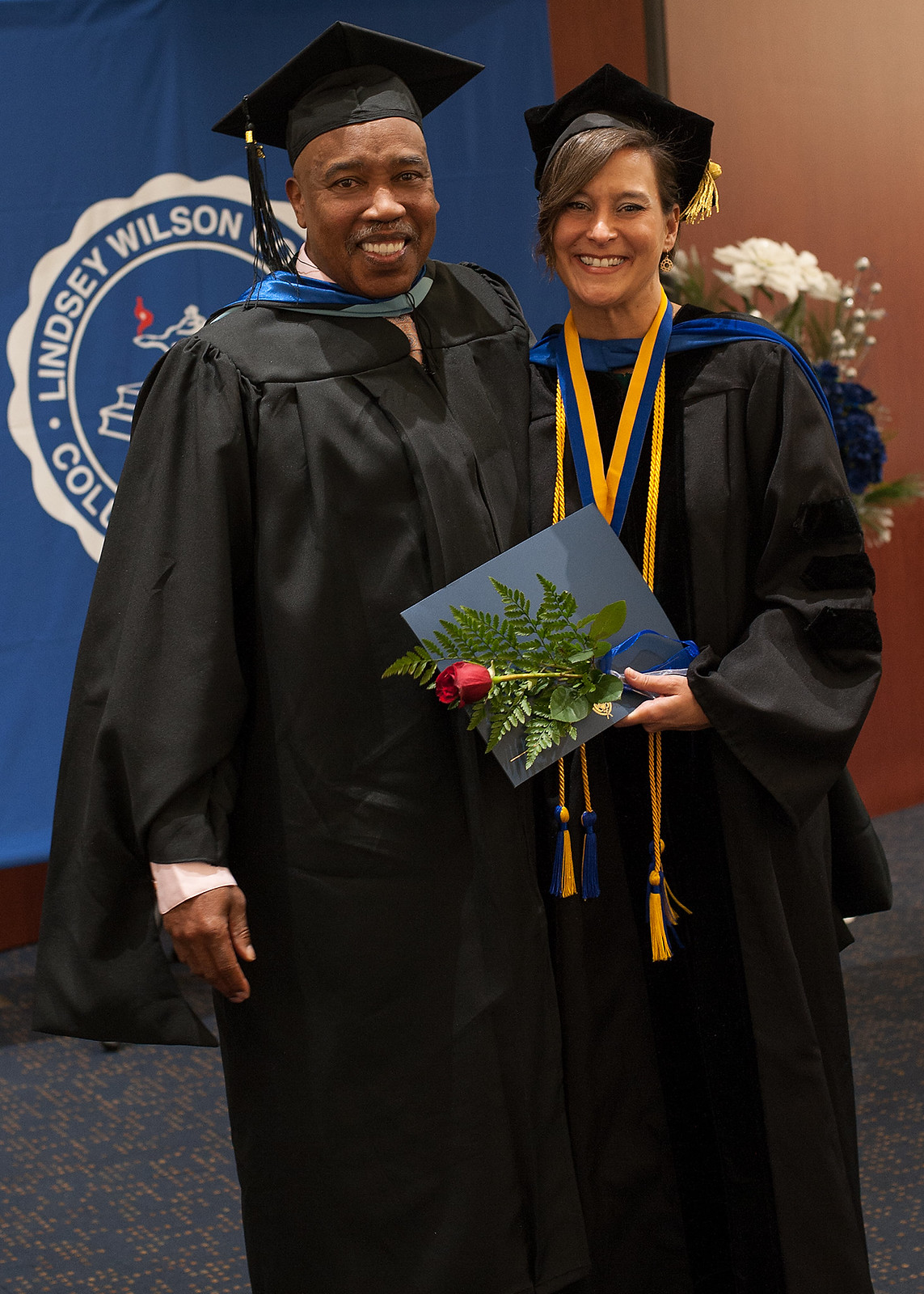This photograph captures a joyful moment of two graduates standing and posing together indoors. The man on the left, with dark skin, wears a black graduation cap, a black robe, and a blue sash draped around his neck. He is smiling warmly at the camera, with his arm affectionately around the woman next to him. The woman, who has dark brown hair, is similarly attired in a black graduation cap and robe, complemented by blue and gold tassels and a blue and gold ribbon around her neck. She holds a blue certificate and a red rose in her hands. Both are grinning proudly at the camera. They stand closely together in front of a blue banner that reads "Lindsey Wilson College," and the backdrop includes a mix of blue and brown flooring and walls, with a bouquet of white and blue flowers visible in the back right corner. The image radiates celebration and accomplishment.